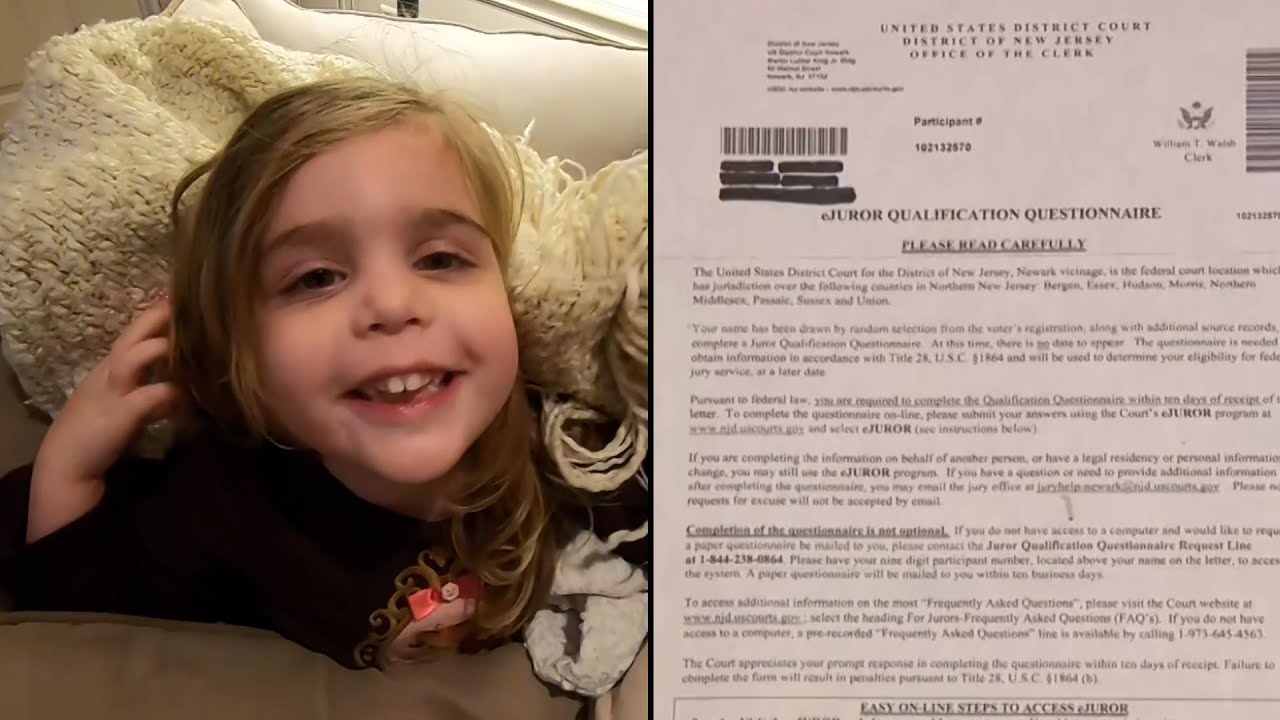The image features a split screen with two distinct sections. On the left side, there is a portrait of a young girl, approximately three to four years old, with dirty blonde, almost light brown hair and brown eyes. She is comfortably nestled on a couch, draped in a fluffy white blanket that resembles a scarf-like material. Behind her is a cream-colored cushion, enhancing her cozy setting. She is wearing a black shirt adorned with a decorative bow. Her youthful face displays mostly grown-in teeth, including two prominent buck teeth. 

On the right side of the image, there is an official document titled "United States District Court, District of New Jersey, Office of the Clerk" with a juror qualification questionnaire. This form, which is mandatory and not optional as stated on the paper, includes details like a participation number and the clerk's name, William T. Walsh, located in the top-right section. The document outlines steps on how to access an EJER account for juror qualification, emphasizing its official and compulsory nature.